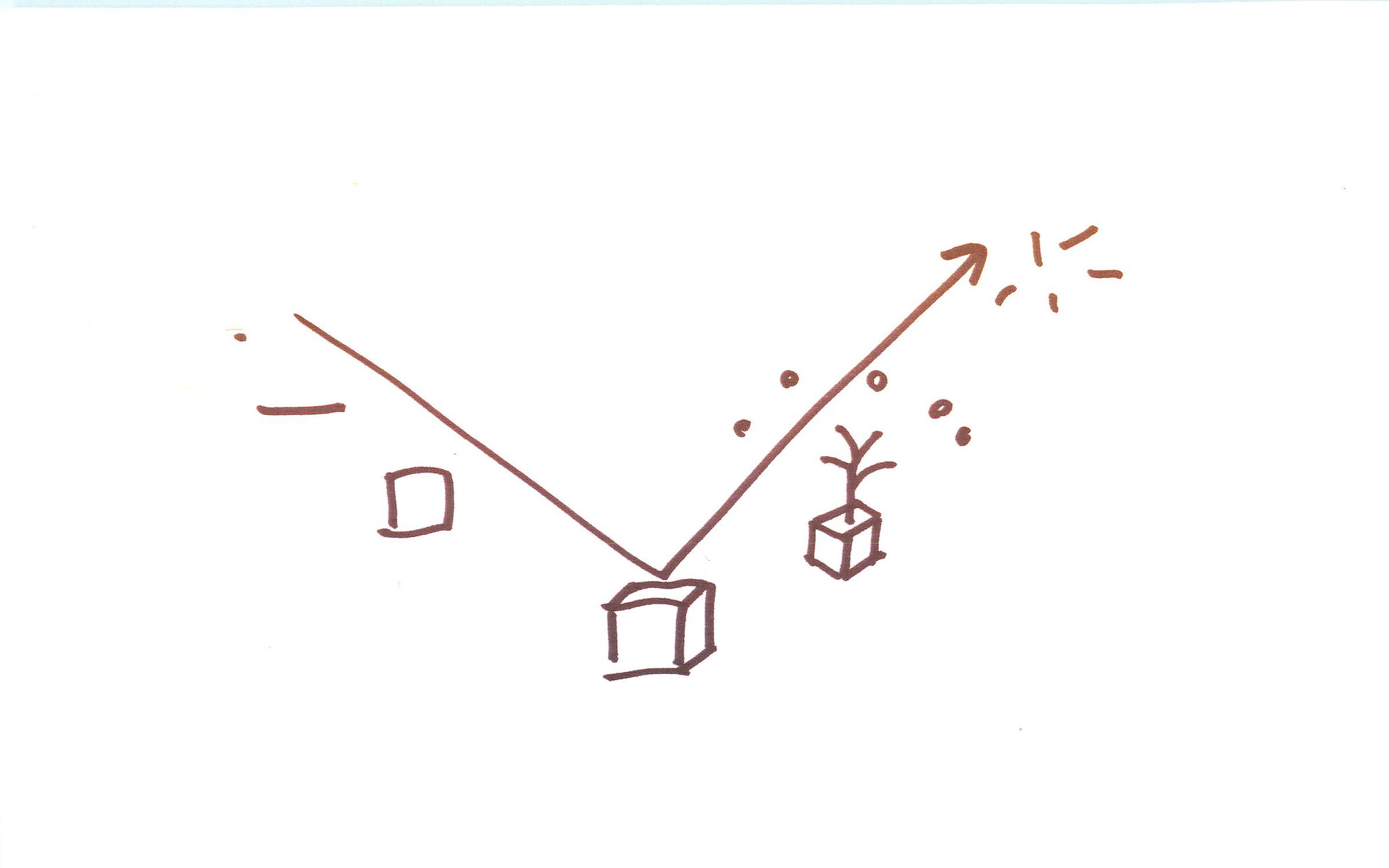This is a detailed hand-drawn image created using a reddish-brown marker. The composition features two intersecting lines forming a 'V' shape. An upward-pointing arrow extends from the right line of the 'V'. Near the top of this arrow, a series of lines that resemble rays emanate from a circular shape, which could be interpreted as a sun.

The image begins in the lower left corner with a small dot, leading to a vertical line that transitions into a three-dimensional box located where the two lines of the 'V' meet. This box is drawn in a darker hue compared to the rest of the elements. Emerging from the box is a tree-like figure comprising a central trunk with multiple branches. 

Encircling the entire image, a series of dots are arranged in a semi-circular pattern, extending outward from the tree and the supposed sun, creating a sense of movement and connectivity between the elements. The background is left blank, providing contrast that highlights the intricate details of the illustration. The image contains no labels or text to provide additional context or explanation.